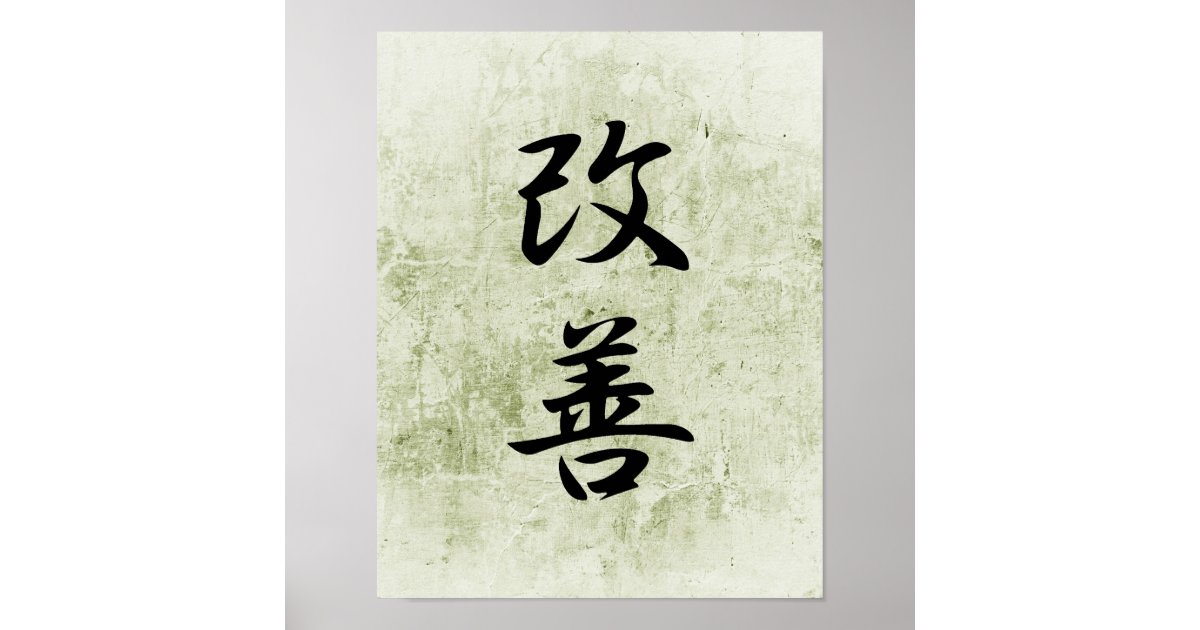The artwork showcases an intricate piece of calligraphy featuring Chinese characters, presented in a vertically oriented rectangular format. Set against a medium grey background, the main focal point is a tan piece of paper that appears weathered and marked with green smudges. The calligraphy itself is composed of clear black strokes, creating a striking contrast with the mottled green and light grey hues beneath it. The upper section of the calligraphy features two characters: one resembling a "Z," and another akin to a "J" with a slash through it. Below these, a longer, more complex character stretches vertically down the center, vaguely reminiscent of a number seven, with additional elements that include a couple of vertical lines, a thick slash, and a fragmented "D"-like shape. The harmonious blend of the tan, green, and grey background highlights the elegant and intricate nature of the black Chinese characters, making the entire piece both visually appealing and thought-provoking.